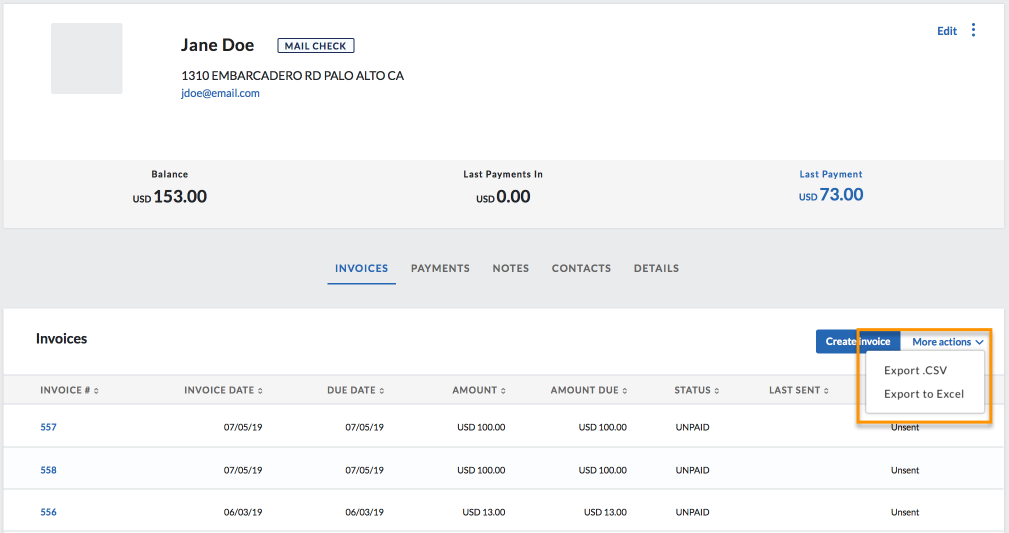In the upper left-hand corner of the image, there is a small gray square with nothing inside it. Adjacent to the square, the name "Jane Doe" is written in black, followed by the number “1310” underneath. Next to these is an address written as "Embarcadero Rd, CA" (California). Under the address in blue text is the email "jdoeatg.email.com." On the right-hand side, the word "Edit" is displayed in blue along with three blue circles.

The background features a light gray border running across the image. On the left side of the section, the word "Balance" is written in black text, with "USD" in capital letters directly beneath it. Beside "USD," the amount "153.00" is displayed. Following some space, the phrase "Last Payment In" appears, with "USD 0.00" below it. On the right-hand side, "Last Payment" is written in blue, followed by "USD" in all capital letters underneath it, and next to it is "73.00."

The section is divided by a darker gray border. Below this, there are different clickable types or tabs: the first one, labeled "Invoices," is underlined in blue, while the subsequent tabs – "Payments," "Notes," "Contacts," and "Details" – appear in dark gray text. The word "Invoices" is also written in black text.

Further, in gray text, "Invoice Number" is indicated with following numbers in blue: "557-558-556." Below each number, the "Invoice Date" is listed in black as "07-05-19," "07-05-19," and "06-03-19," respectively. The "Due Date" column mirrors the invoice dates. The amounts "USD 100.00, 100.00" and "13.00" are shown under "USD Amount," followed by the respective due amounts which match exactly. The "Status" column displays "Unpaid" for all listings.

At the bottom, there is a box with an orange square border containing the options to "Export.csv" and "Export to Excel" in black text.